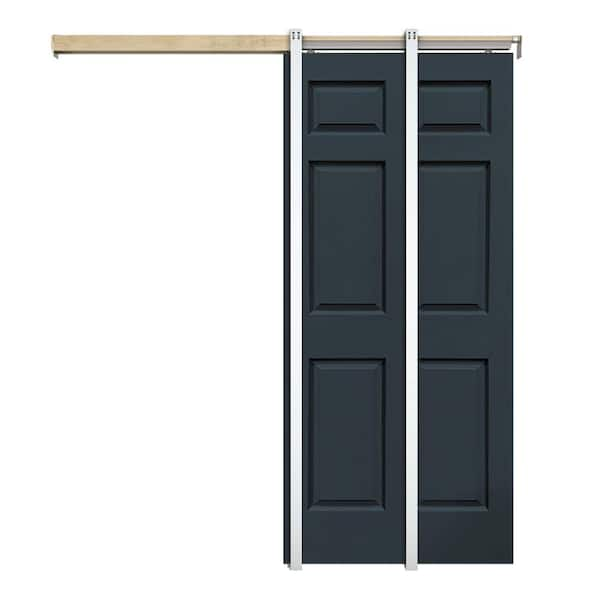This image depicts a modern, digitally created black door with a unique design. The door, reminiscent of a barn door style, is attached to a wooden top rail of a light wood color, situated on the right-hand side. This top rail is connected to vertical silver metal tracks that run down its length, giving the appearance that the door could fold into itself. The door features three rectangular vertical patterns, adding to its distinctive look. There is a white background and a white wall on one side, with a white railing or border running alongside the door from top to bottom. No text or people are present in the image.